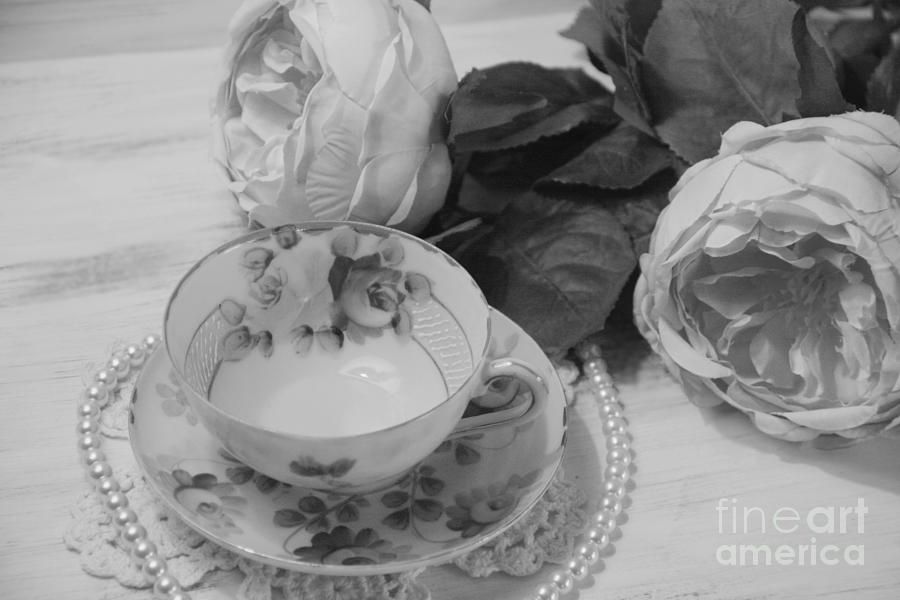This black and white photograph appears meticulously arranged, featuring a delicate tea set and floral elements on a flat surface. The focal point in the lower left is an ornate teacup with matching floral designs on both the cup and its saucer. This elegant duo rests on a small white doily. Encircling the saucer is a string of pearls, adding a layer of refinement. To the right, two large flowers, possibly roses or carnations with accompanying leaves, partly cover the pearls and extend under the saucer. The flat surface underneath could be wooden or marble, contributing to the photo’s textured backdrop. Dominating the bottom right corner is the text "Fine Art America," subtly branding this carefully composed shot. Overall, the image exudes an air of sophistication and timeless elegance, well-framed from a downward angle, capturing both detail and depth.